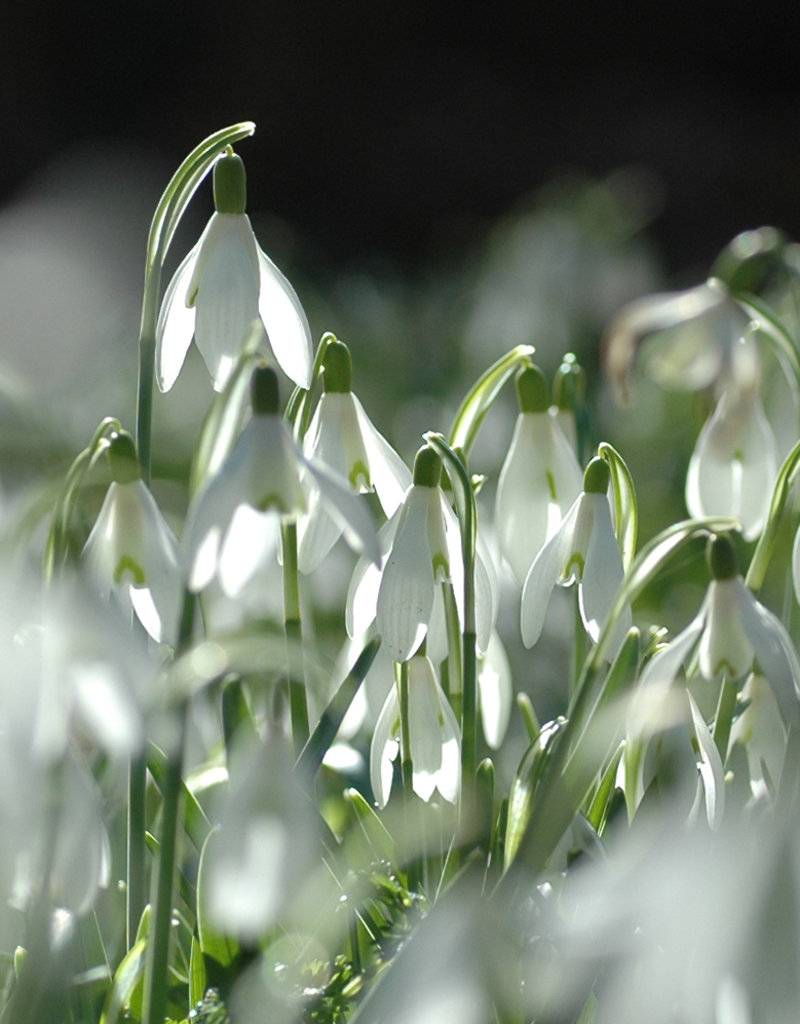The image is a close-up of a field brimming with white flowers, specifically focusing on their delicate structure. Each flower, perched on a slender green stem that stretches upwards, features petals that gracefully droop downwards, creating a lampshade effect. The background is purposefully blurred, fading into vague black and white shapes, drawing full attention to the central and forefront flowers. Though the petals generally appear in clusters of three, some cluster in groups of four to five, hanging down from their stems. This deliberate fade effect emphasizes the flowers in the foreground, highlighting their detailed, downward-facing petals against the otherwise indistinct backdrop. The image is devoid of text, leaving the pure, natural beauty of the white and green flowers uninterrupted.